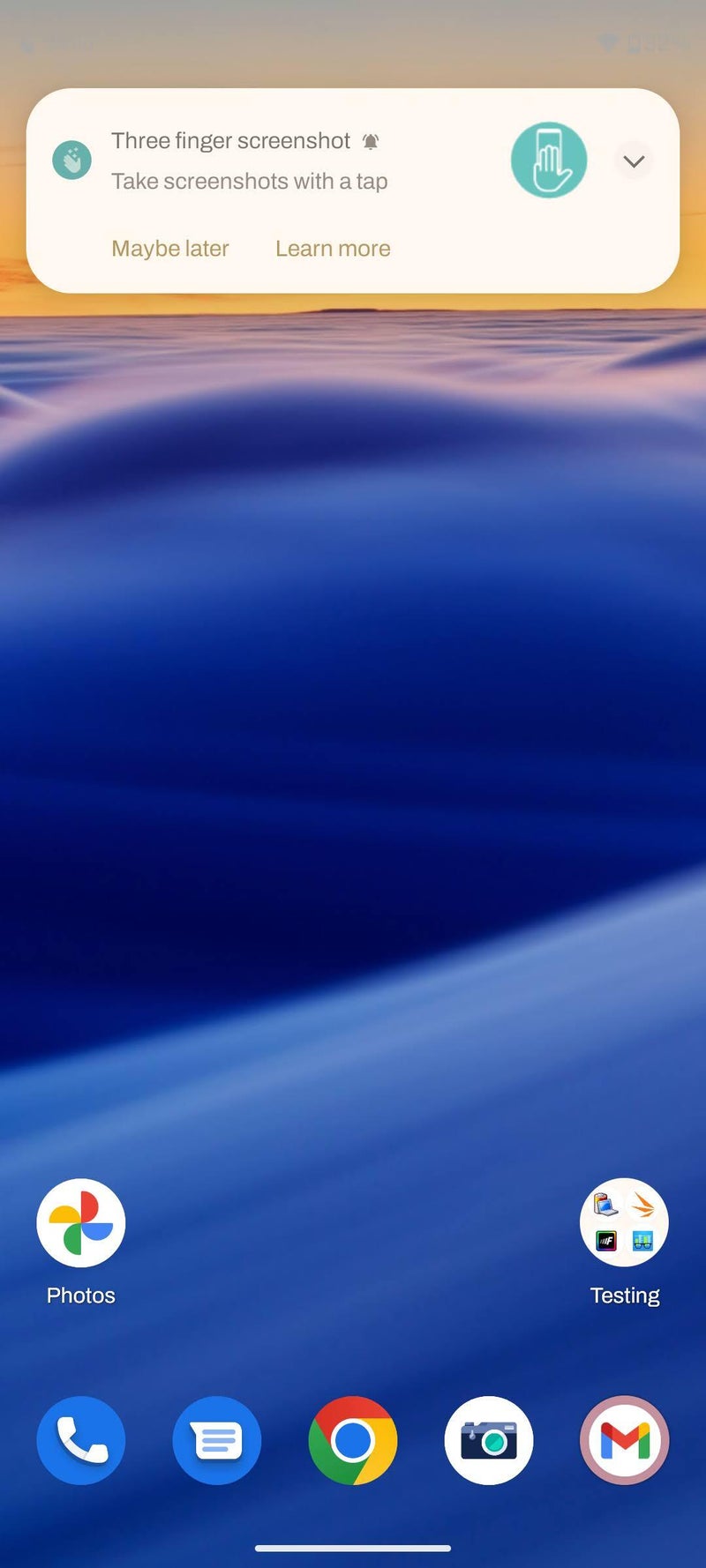A smartphone screen featuring a gradient background that transitions from gray-brown at the top to gold. Overlaid on this background is a white pop-up notification with a green icon displaying a white cell phone with three fingers on it. The notification text reads: "Three-finger shot, bell, notification. Take screenshots with a tap," followed by the options "Maybe later" and "Learn more." Below this, the background transitions to stylized blue water. At the bottom, there are icons for Photos (Google Photos app), Testing, Call, Text, Google, and another app represented by an 'M' with Google colors. The screen displays a range of colors including blue, green, yellow, red, brown, white, black, and orange. Notably, there is no status bar or indication of the top information typically found on a cell phone screen.